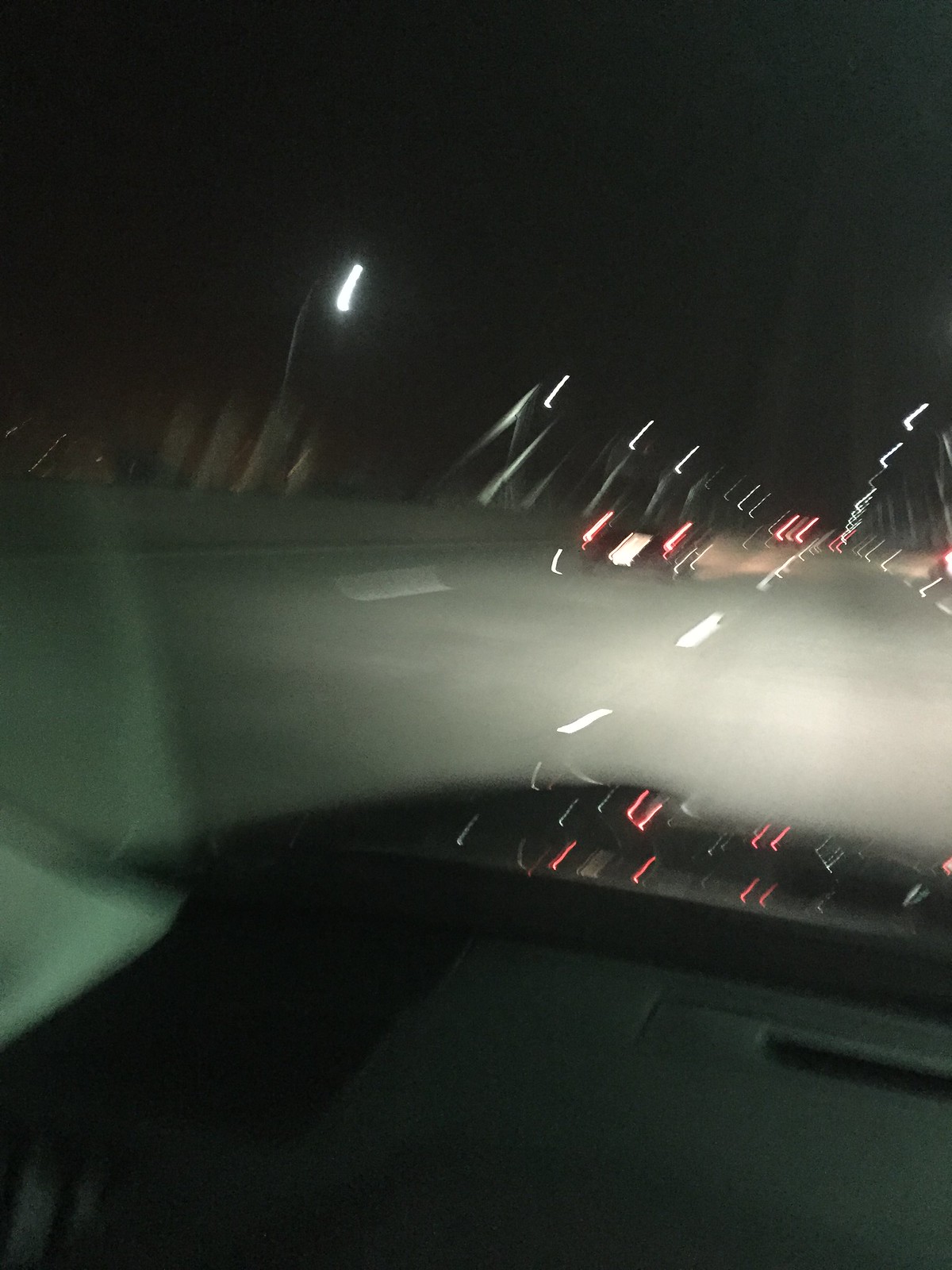A captivating photo taken from the interior of a moving vehicle at night. The dark gray dashboard is visible in the lower section of the image, framing the dynamic scene. The vehicle is in motion, evident from the beautifully blurred surroundings that create a sense of speed. The middle section of the image features a hazy, smoky line of light that illuminates the road ahead, revealing the dark blacktop and faint white lane markings. The upper part of the image is dominated by a pitch-black night sky punctuated by lamp posts, whose lights appear as small, white streaks. Adding to the complexity, the scene is adorned with numerous pinkish lines, likely the blurred brake lights of other vehicles ahead. Some of these lines might also be reflections in the windshield, adding layers to this mesmerizing nighttime journey.